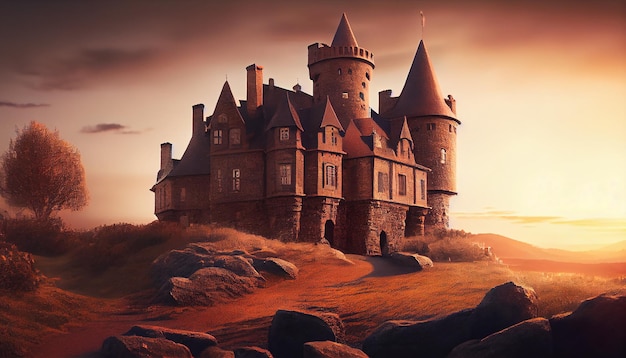The image depicts a large, medieval-style castle made of brown bricks, standing majestically in the center. This imposing structure has at least three stories and features two prominent, arch-shaped entrances. The castle is characterized by numerous pointy, triangular tops and includes two cylindrical structures near its right side. It is adorned with many windows on its second and third floors, adding to its intricate detail. The ground surrounding the castle has a brownish and burnt orange hue, littered with large stones and boulders, lending an eerie, desolate feeling to the scene. On the left of the image, a lone brown tree with some sparse, yellowish foliage stands in stark contrast to the castle. The sky is a blend of dark grey at the top, transitioning to a bright yellow towards the right, evoking the sense of either a sunset or sunrise, which casts an ethereal glow over the entire scene. The artwork emanates a surreal, almost otherworldly atmosphere, emphasizing the solitary and mysterious nature of the castle.